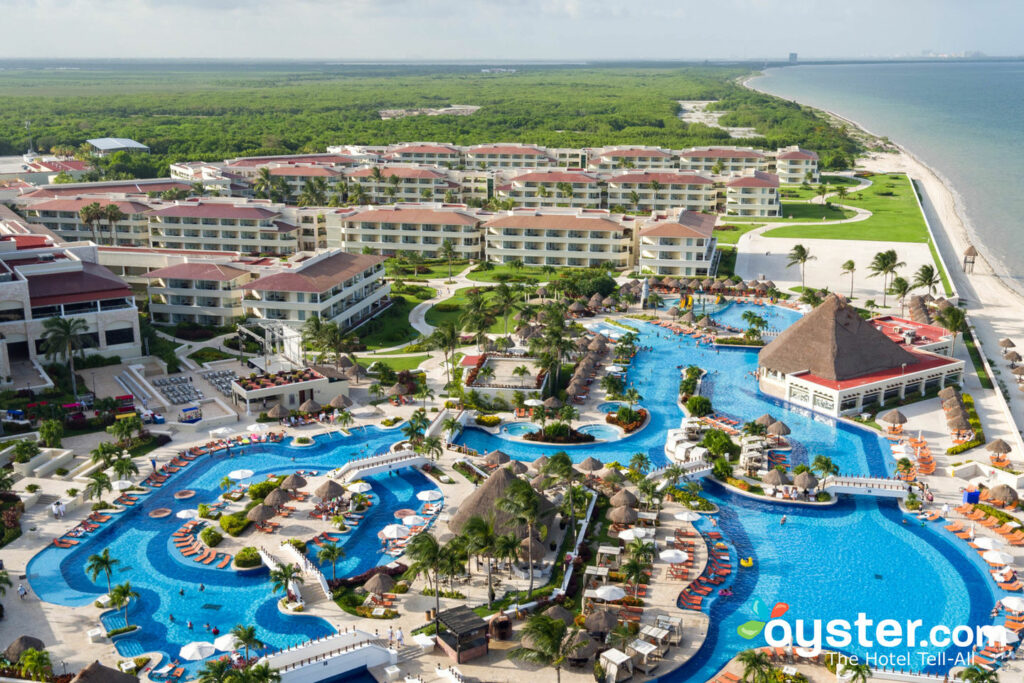The image, an advertisement for Oyster.com's Hotel Tello, showcases a breathtaking bird's-eye view of a sprawling resort located on the beach in Florida. Dominating the foreground, a vast Lazy River Pool snakes around the resort, dotted with man-made islands, floating bars, and lounge chairs aplenty, creating an inviting sanctuary for relaxation. The resort itself features multiple rows of hotel buildings surrounded by lush greenery, including a grassy field or swamp area, giving way to a large cityscape seen in the distant background. Enhanced with a high level of detail, this striking computer-generated image encapsulates the allure of an opulent, family-friendly tourist destination. The "Oyster.com" logo with "Hotel Tell All" appears in white text at the bottom of the image, adding a finishing touch to this dream-like vacation spot.